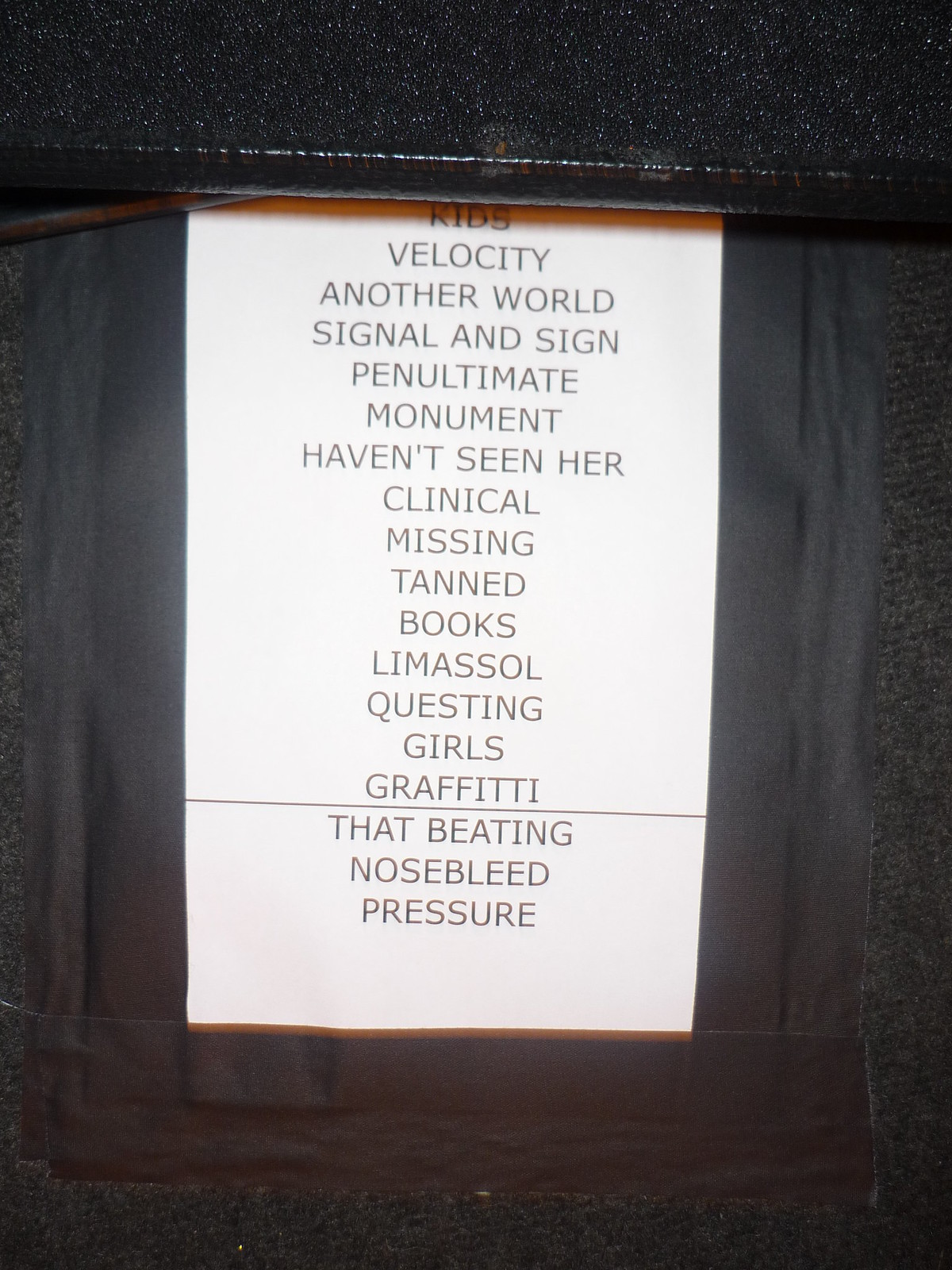The image features a white piece of paper with black, typed text laid on a black stage. The paper, likely a setlist for a band's performance, is taped at the bottom to the stage floor. The setlist is organized from top to bottom and contains the following song titles: "Kids," "Velocity," "Another World," "Signal and Sign," "Penultimate," "Monument," "Haven't Seen Her," "Clinical," "Missing," "Tanned," "Books," "Limassol," "Questing," "Girls," and "Graffiti." Approximately two-thirds down the list, a black line separates the main set from the encore. Below this line, three encore songs are listed: "That Beating," "Nosebleed," and "Pressure." All the text is written in block capitals, providing a clear and organized guide for the band.